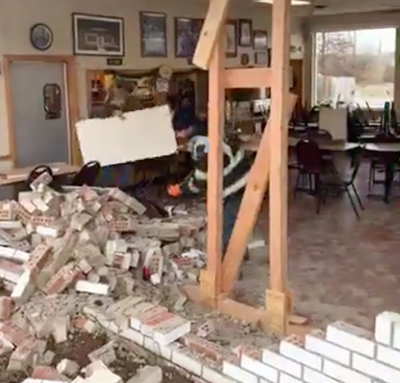The image depicts the interior of a partially demolished restaurant currently undergoing renovation. In the foreground, a large portion of a brick wall has been destroyed, with the rubble spread out into the room. The wall's remnants include white bricks mixed with reddish-orange bricks, while some still remain partially stacked on the right side. Prominently, a fresh wood support beam, constructed from two-by-fours, stands in the middle of the space, suggesting ongoing structural work.

The restaurant features a series of tables and booths, with framed pictures adorning the cream-colored walls. A gray door on the left side hints at an entry into a different section of the building, possibly a kitchen. The large window at the back of the room offers a view of a lawn, trees, and the skyline beyond, bringing natural light into the space.

In the semi-completed building, exposed wood and bricks hint at the construction effort. Visible in the blurry background is a worker, identifiable by their orange gloves and hat, actively engaged in the renovation work.